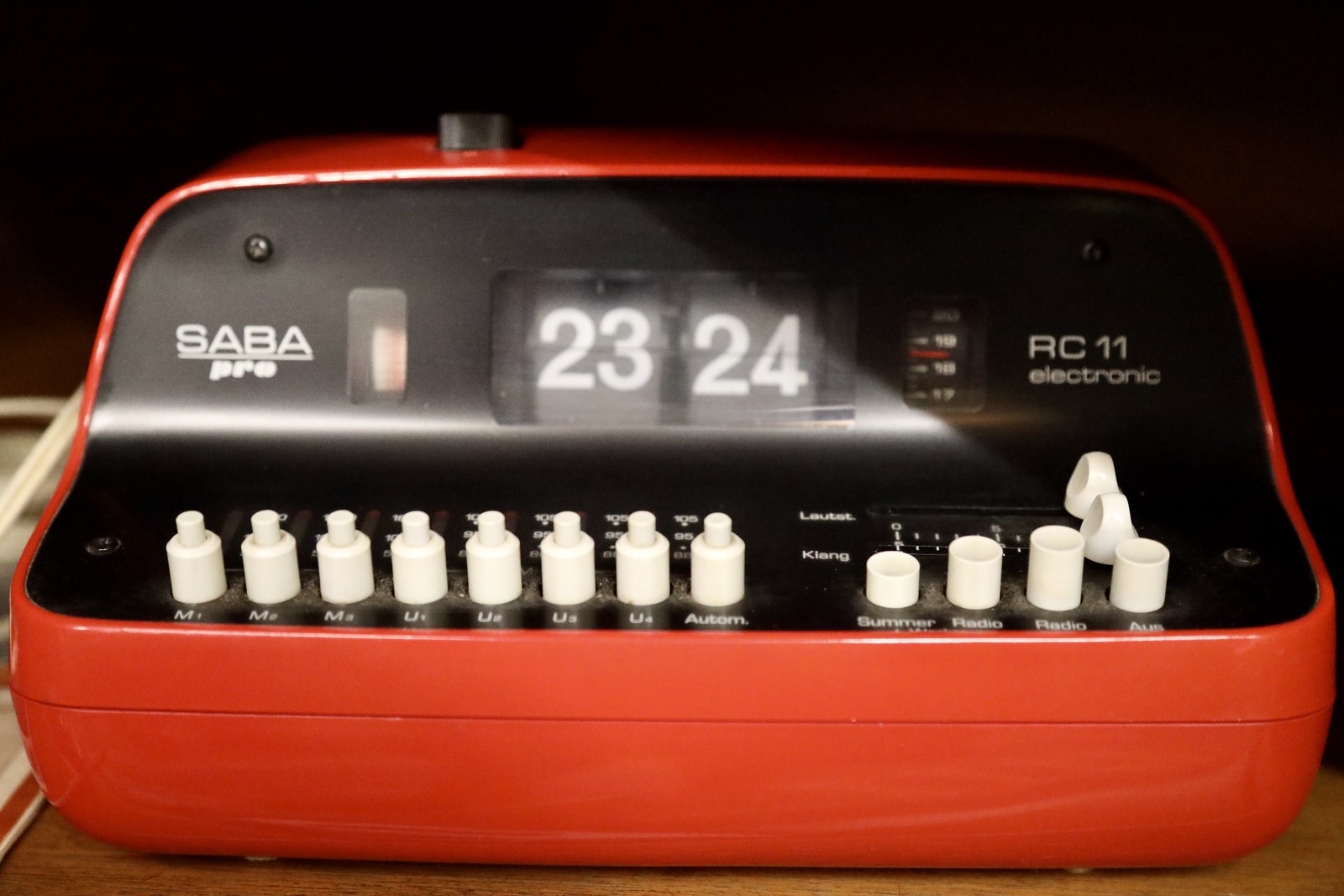This is an image showing a close-up view of a vintage electronic radio, prominently featuring a blend of black and orange elements with several white knobs and buttons. The radio has a distinct design with a curved black top section and a vibrant orange bottom. On the left side of the black surface, the text "SABA" is displayed in all caps, followed by "P-R-E" and the numbers "2324," all written in white. The upper right corner of the device also includes the label "R-C-11 electronic."

The interface includes various white knobs and buttons, with labels such as "A-U-S," "radio," and others, though some words are partially cut off. Notably, there are multiple buttons labeled "radio," one larger and one smaller. Additional labeled sections like "A-U-T-O-M," "U4," "U3," "U2," "U1," "M3," "M2," and "M1" suggest functionality for different settings or modes. The foreground features some circular and closely positioned pins, possibly for volume or tuning adjustments, enhancing its intricate and detailed appearance. White tiles marked "L-O-U-T-A-T" and "K-L-A-N-G" add to the complexity of the control panel, providing an insightful snapshot of the radio's accessible features.